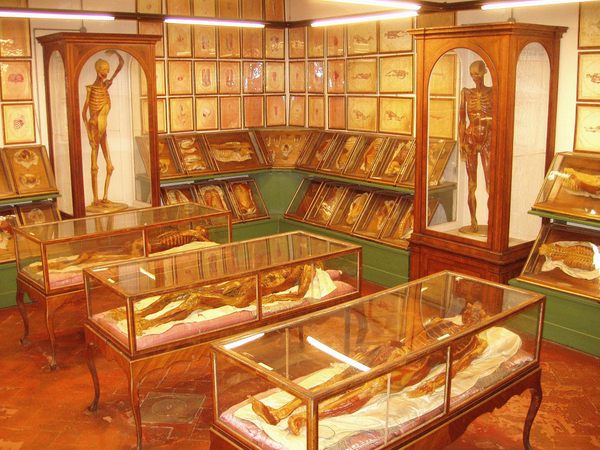The illustration depicts a museum exhibit room dedicated to skeletons and fossils. The room features an orangish-brown tile floor with sections of green paint on the lower portions of the walls. Two tall, glass-windowed display cabinets showcase human skeletons—one standing straight and the other with an arm raised overhead. On the floor, three brown wooden tables hold narrow glass-topped cabinets with skeletons resting atop white pillows and pink satin padding. These coffins are aligned in a row from the center-right to the left side of the image. The room also has brown wooden and glass curio cabinets containing additional human skeletons. The walls are adorned with framed pictures and mounted skeletal remains of various animals, including noticeable fish fossils. The lighting casts a warm amber glow, enhancing the display of meticulously preserved bones and body parts, set against a backdrop of predominantly yellow, gold, and orange hues. The exhibit appears to be dedicated to medical research and education.